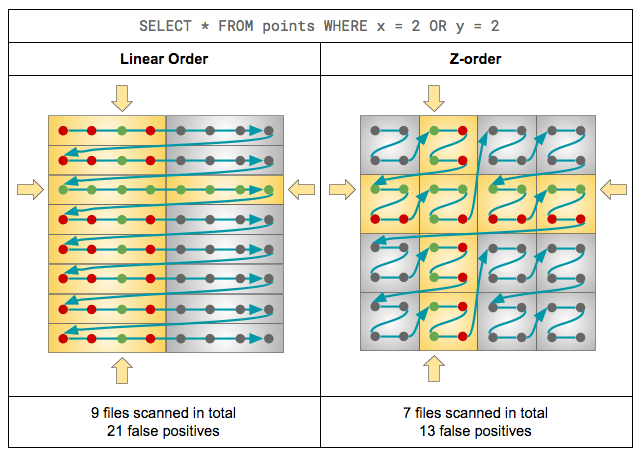The image features a detailed diagram illustrating two distinct methods for implementing an SQL query, with a clear comparison between "Linear Order" and "Z Order." The top of the poster displays the syntax "SELECT * FROM POINTS WHERE X = 2 OR Y = 2." Below this heading, the diagram is divided into two parts. On the left side, labeled "Linear Order," the background is split with half in yellow and the other half in grey. This section contains numerous red and green dots connected by blue lines with arrows pointing toward the center. It is noted at the bottom that "9 files scanned in total, 21 false positives." On the right side, labeled "Z Order," the diagram is characterized by boxes with a Z-shaped pattern, integrating yellow crosses within grey boxes and yellow arrows within them. The bottom text indicates "7 files scanned in total, 13 false positives." The diagram visually emphasizes the differences in file scanning efficiency and accuracy between the two methods, hinting at reduced false positives with the Z order compared to linear order.